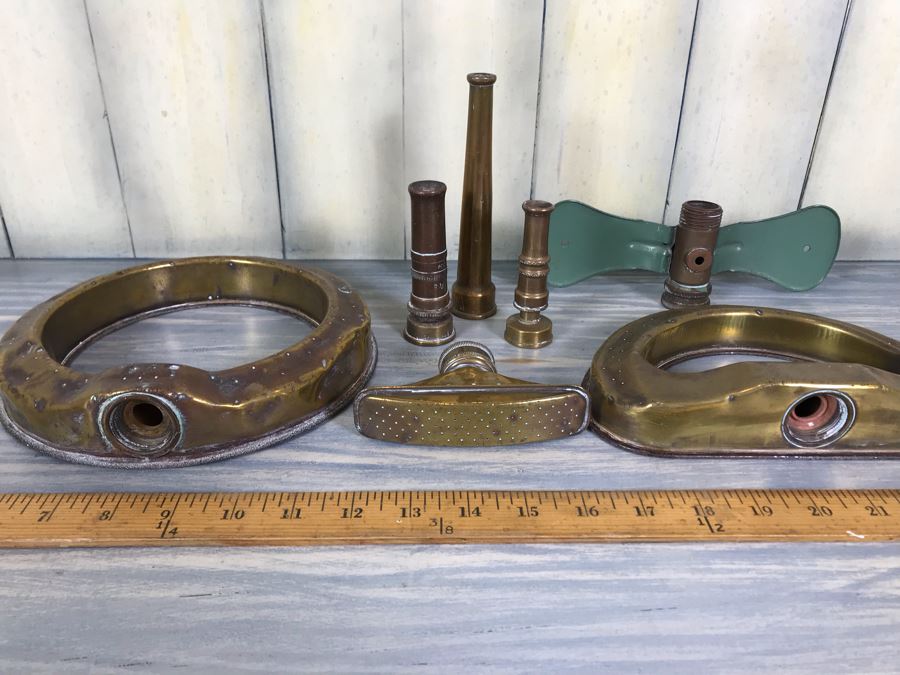This detailed full-color, well-lit indoor photograph depicts an arrangement of polished brass instruments and tools on a light gray, wood grain table. The table features a horizontally placed wooden ruler marked clearly from 7 to 21 inches, partially cut off at the bottom edges of the square image. Against a vertically planked white wall, the objects appear to be neatly organized, as if for sale or display.

To the left, there is a large cylindrical brass piece with a round hole at the bottom, possibly designed for attachment to other components. Near this, a smaller brass piece with a curved base and threaded top might connect to the larger part. Above, closer to the wall, three upright, tube-like brass pieces form a row. The left one is short and uniform in diameter, the middle one tapers upward, and the right one is the smallest, with a base that narrows as it rises.

In the center, touching the wall, a cylindrical brown piece flaunts two green blades resembling lawnmower parts or similar equipment. On the right side, below this cylindrical object and just above the ruler, lies a bronze piece with a half-circle shape, which mirrors the piece on the left but is halved and horizontally straight at the bottom with a round opening.

These various metal pieces, potentially hose parts or saddlery components, suggest functionality and versatility, displayed meticulously to single out their distinct structures and pristine polished surfaces.